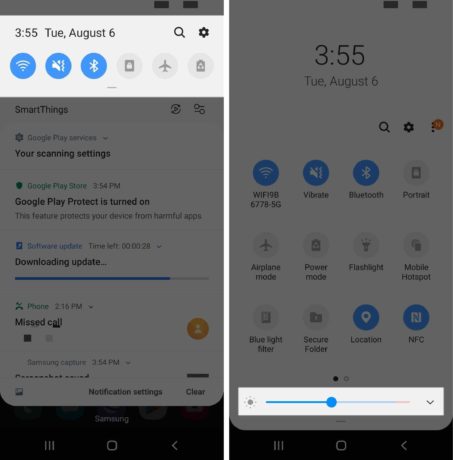**Detailed Image Description:**

The image is a collage of two screenshots captured from a smartphone, both showcasing various settings and notification details.

**Left Screenshot:**
At the top of the screenshot, the status bar displays the current time, "3:55", and the date, "Tuesday, August 6th". The bar also includes icons for Wi-Fi signal strength, a mute notification, Bluetooth connectivity, and Airplane Mode, among others.

Beneath the status bar, a dark gray filter theme is applied to the notifications and settings panel. The following sections and notifications are visible in this area:

- **SmartThings**: Indicating the presence of connected smart devices.
- **Google Play Services**: Likely prompting for updates or notifications.
- **Scanning Settings**: Options related to scanning functionalities on the smartphone.
- **Google Play Store**: The main hub for downloading and updating apps.
- **Google Play Protect**: A security feature that actively protects the device from harmful apps.
- **Software Update**: A notification regarding an ongoing or pending software update.
- **Downloading Update**: Indicates that a software update is currently being downloaded.
- **Phone Missed Call**: Alerts the user of a missed phone call.
- **Samsung Capture**: Indicates a screenshot or screen capturing application.
- **Notification Settings**: An option to modify how notifications are received and displayed.

**Right Screenshot:**
This screenshot also features a dark-themed interface and appears to be the settings panel for adjusting the phone's brightness. The brightness slider is near the halfway mark. Visible in this panel are various icons for quick settings, including:

- **Wi-Fi**: Status of the Wi-Fi connection.
- **Vibrate**: Indicates whether the phone is set to vibrate mode.
- **Bluetooth**: Status of the Bluetooth connection.
- **Portrait Mode**: Likely the screen orientation setting.
- **Airplane Mode**: Quick access toggle for airplane mode.
  
Both screenshots collectively illustrate the user navigating the quick settings and notification panel of their smartphone, providing an overview of ongoing processes and connectivity statuses.